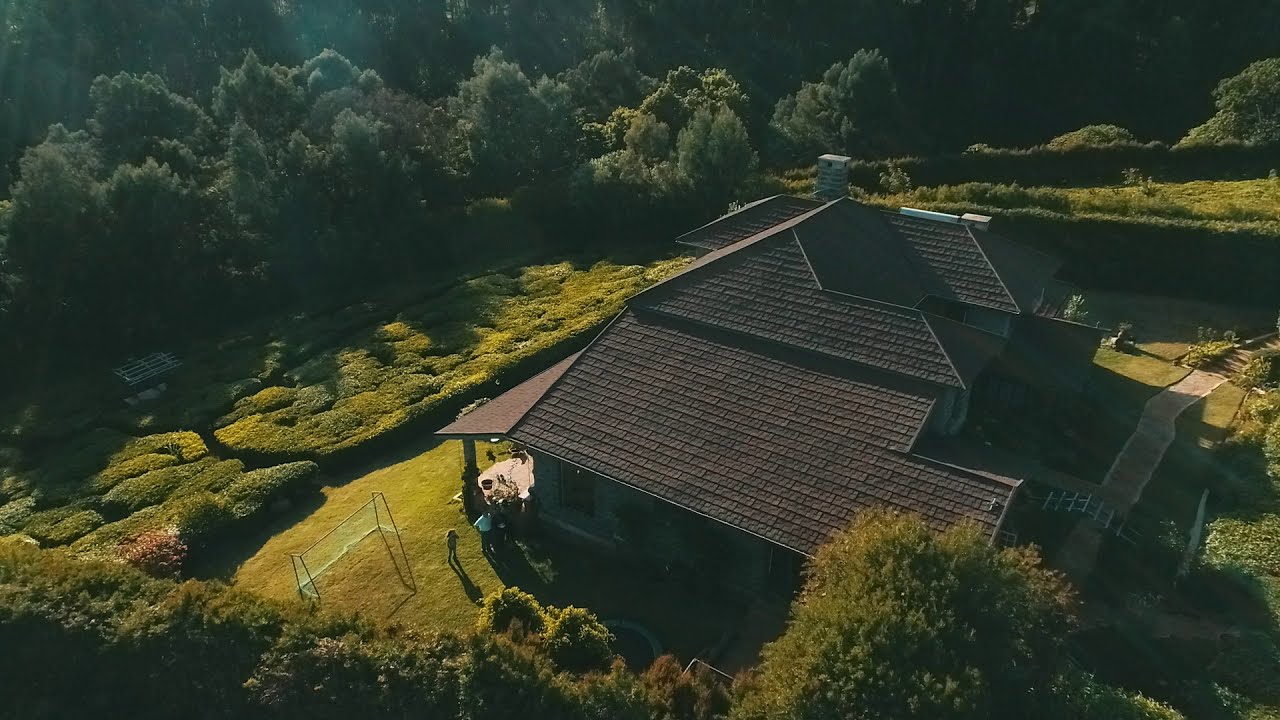This aerial photograph captures a substantial modern house set in the countryside, surrounded by lush greenery. The house, prominently positioned near the center of the image, features a sloped, shingled roof with multiple levels and a brownish hue. A chimney stands tall among the other roof structures. Surrounding the house is a meticulously manicured lawn, bordered by dense woods with tall trees, low-lying bushes, and various shrubs.

In the backyard, several elements stand out: a soccer goal and a trampoline are visible on the neatly cut grass. There are multiple people in the yard, including a child and two adults, casting long shadows suggesting the photo was taken early in the morning or late in the afternoon. The photo, taken from a high vantage point possibly with a drone, shows no text and is rich in colors like green, brown, orange, yellow, tan, and gray.

Overall, the house exudes a sense of grandeur and affluence, featuring a porch-like canopy structure supported by poles. Despite the detailed roof and yard, it's somewhat challenging to determine from the aerial perspective whether the visible porch is at the front or the back of the house. The upper portion of the image is shaded by the numerous surrounding trees, emphasizing the house's secluded, picturesque setting.